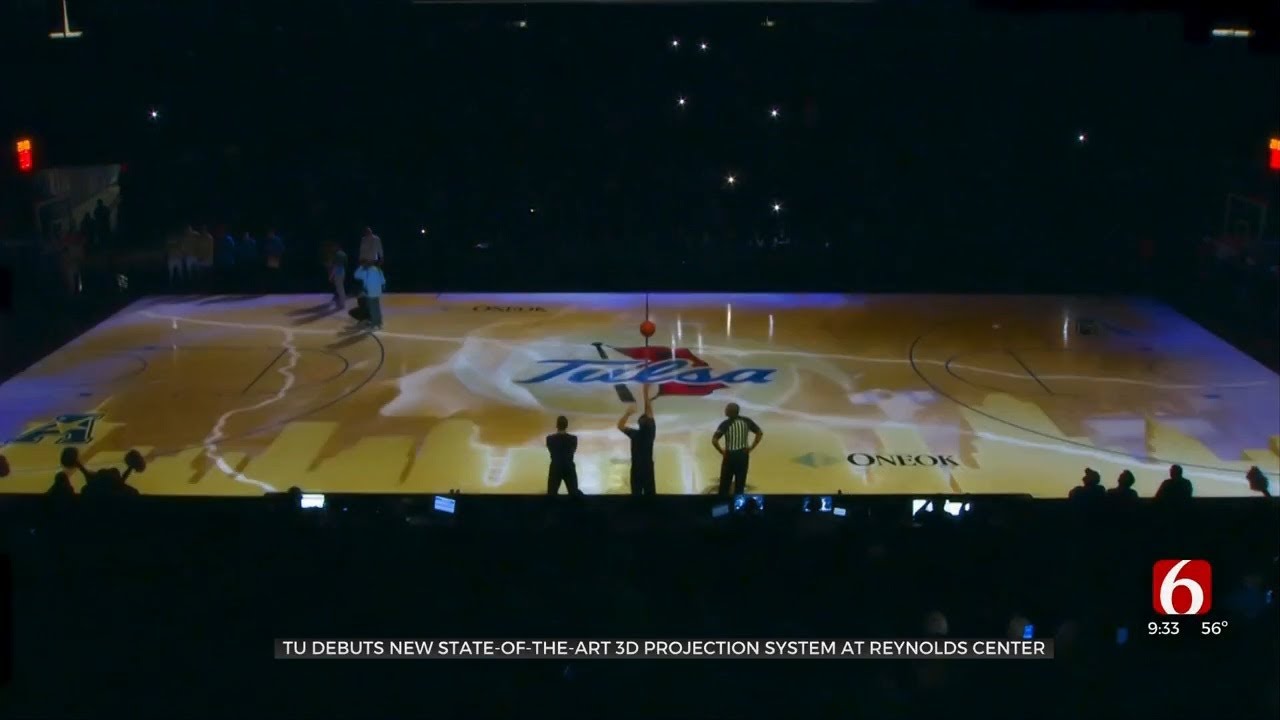In this photograph, presented by Channel 6 News, we see a darkened arena that appears to be the Reynolds Center at Tulsa University, showcasing their new state-of-the-art 3D projection system. The basketball court is illuminated, contrasting sharply with the pitch-black grandstands surrounding it, except for a few specks of light from attendees' cell phones. The court itself has a light background with "Tulsa" prominently displayed in blue at its center. On the bottom center and right side of the court, there are several figures: three men, two in black and one in a referee's outfit, with the middle man tossing a basketball into the air. Additional referees and basketball players are seen preparing on the sidelines, ready to engage. The image includes a black banner with white text at the bottom, reading, "TU debuts new state-of-the-art 3D projection system at Reynolds Center," and features the Channel 6 logo—a red square with a white number six—and the current time and temperature: 9:33 p.m. and 56 degrees.